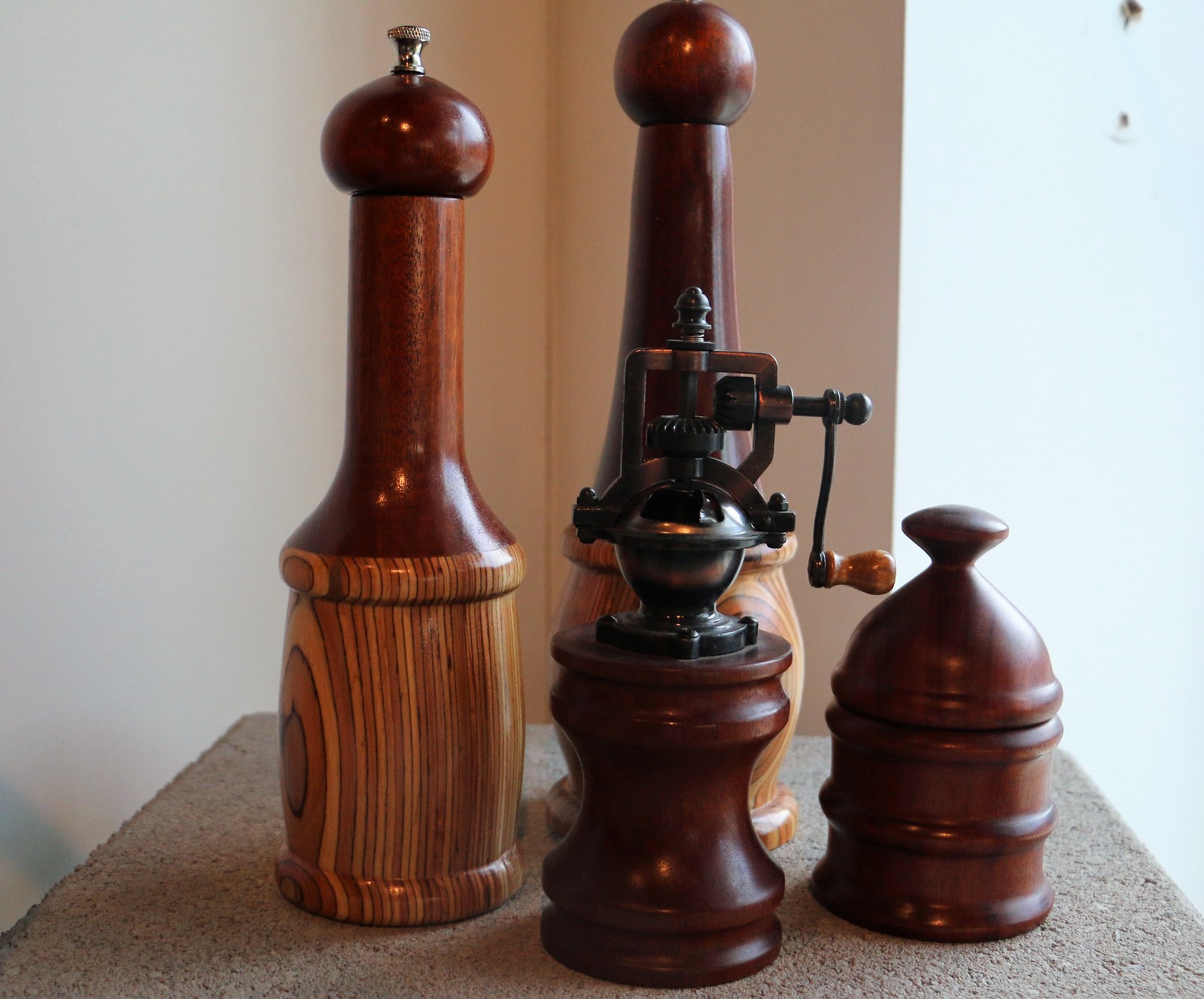The photograph showcases a collection of four distinctive pepper grinders, all primarily crafted from dark brown wood and embodying an elegant, yet vintage design. The most prominent grinder in the center features an intricate metal grinding mechanism with a hand-crank that enables a detailed and mechanical process for dispensing pepper, suggesting an old-fashioned, yet sophisticated charm. Flanking this centerpiece are two tall, cylindrical wooden grinders, one with a lighter wood grain pattern at its base. These two appear sleek and simple, with traditional twist-to-grind tops. A fourth grinder, noticeably shorter, also boasts a crank mechanism, albeit less complex than the central one. This collection, despite its antique aesthetics, appears to be in mint condition, hinting at minimal to no usage. They are neatly arranged on a shelf or table against an off-white background, presenting an overall impression of timeless elegance and functionality.